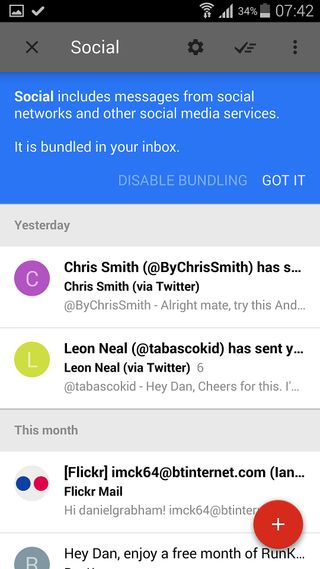This screenshot from a phone presents a detailed view of a notification screen segment. At the very top, a black status bar exhibits several icons including a Wi-Fi symbol, battery indicator, and the time, which reads 7:42. 

Directly underneath, a gray header bar features an 'X' for closing on the far left, a white 'Social' text label, followed by a gear icon, a checkmark with three adjacent lines, and three vertical dots for additional options. Below this header, a blue rectangle states: "Social includes messages from social networks and other social media services. It is bundled in your inbox." There are also options to disable bundling or acknowledge with "Got it."

Following this, the screen labels the preceding updates with "Yesterday," succeeded by a purple circle showcasing the initial 'C' attributed to 'Chris Smith' with the message, "All right, mate, try this." Below, a yellow circle bearing the initial 'L' is associated with 'Leon Neal,' displaying the message, "Hey, Dan, cheers for this."

Further down, a light gray title bar marked with "This Month" categorizes older notifications. Underneath, various advertisements appear. One ad is from Flickr, and another offers a free month subscription, partially readable as "run something" or "run K."